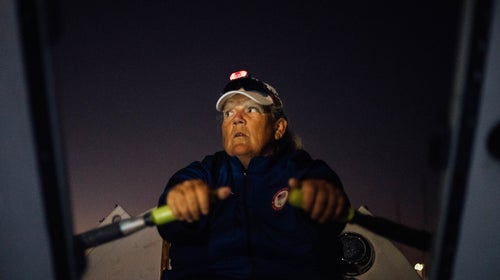The image depicts an elderly woman rowing a boat under a night sky filled with stars. The photo is taken from a low angle, possibly from within the boat itself, providing a view upward towards the woman. She is dressed in a navy blue jacket adorned with a patch featuring the American flag in red, white, and blue on her left breast pocket. Her attire includes a white cap, over which she has mounted a headlamp. The woman's face, tanned and weathered from what appears to be a life spent outdoors, shows signs of distress as she gazes off to the left side of the image. Her hands firmly grip the lime green handles of the yellow-tipped oars, suggesting she is actively engaged in rowing. The surrounding darkness and her intense expression add a dramatic element to the scene, emphasizing the solitary and tense moment captured.